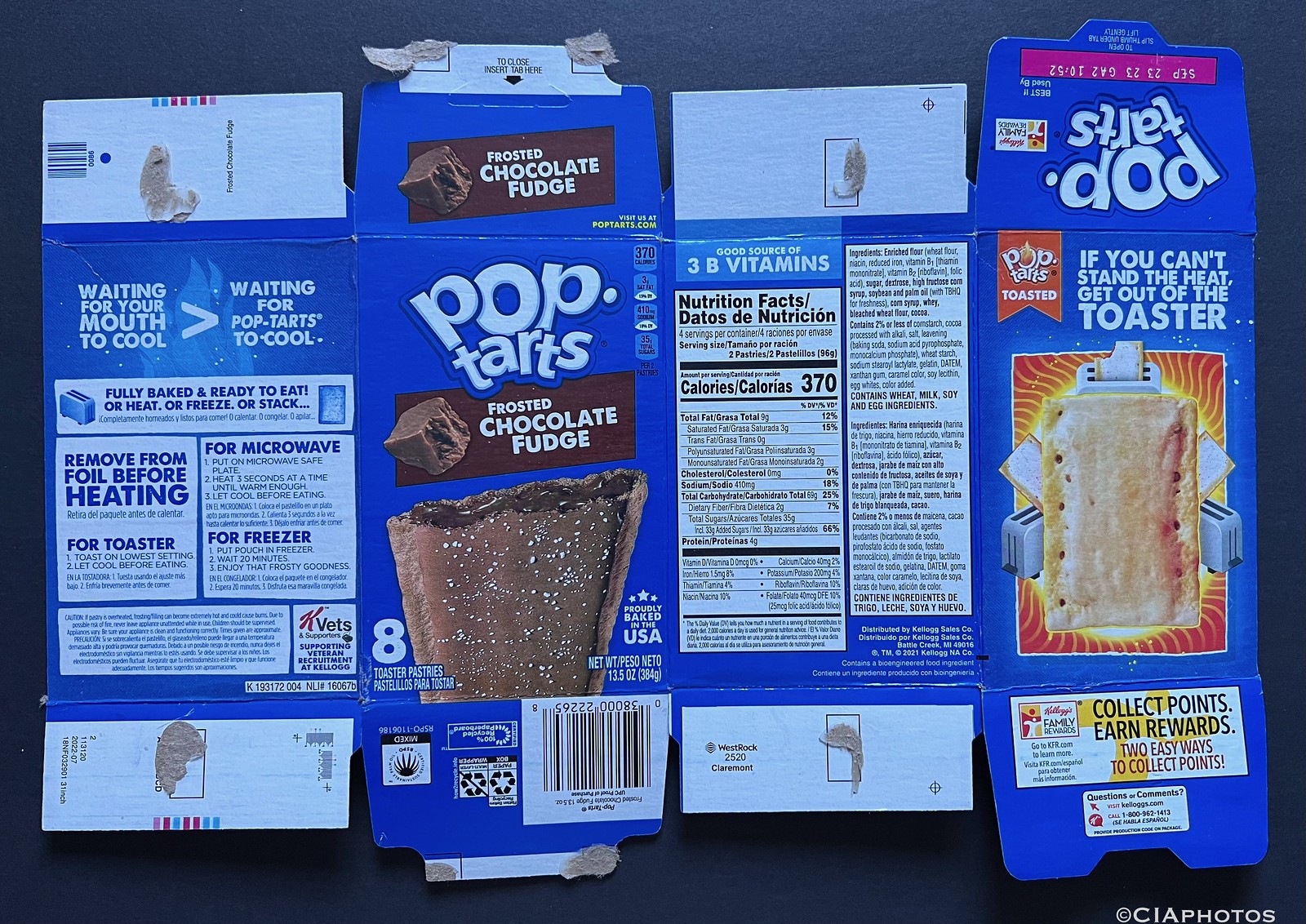This photograph showcases a flattened box of Chocolate Fudge Pop-Tarts. The packaging is predominantly blue and contains multiple elements in white and black font. At the bottom of the image, a white watermark reads "CIA photos." 

The main section of the box displays a picture of a frosted Chocolate Fudge Pop-Tart, with the caption "Frosted Chocolate Fudge" above it in white font. A prominent image of a brown fudge piece complements the branding. The text "8 toaster pastries" is printed in white, indicating the quantity contained in the package. 

One side of the packaging features a typical nutrition label along with the phrase, "If you can't stand the heat, get out of the toaster," in white font. This section also shows a tan Pop-Tart image flanked by two silver toasters. At the bottom, it encourages consumers to "Collect points, earn rewards," and elaborates on "Two easy ways to collect points" in black font.

Another panel contains the playful warning, "Waiting for your mouth to cool, waiting for Pop-Tarts to cool," also in white font. Additional navy text adds further context. 

Overall, the extensive details and vibrant imagery provide a comprehensive look at the Chocolate Fudge Pop-Tarts box.